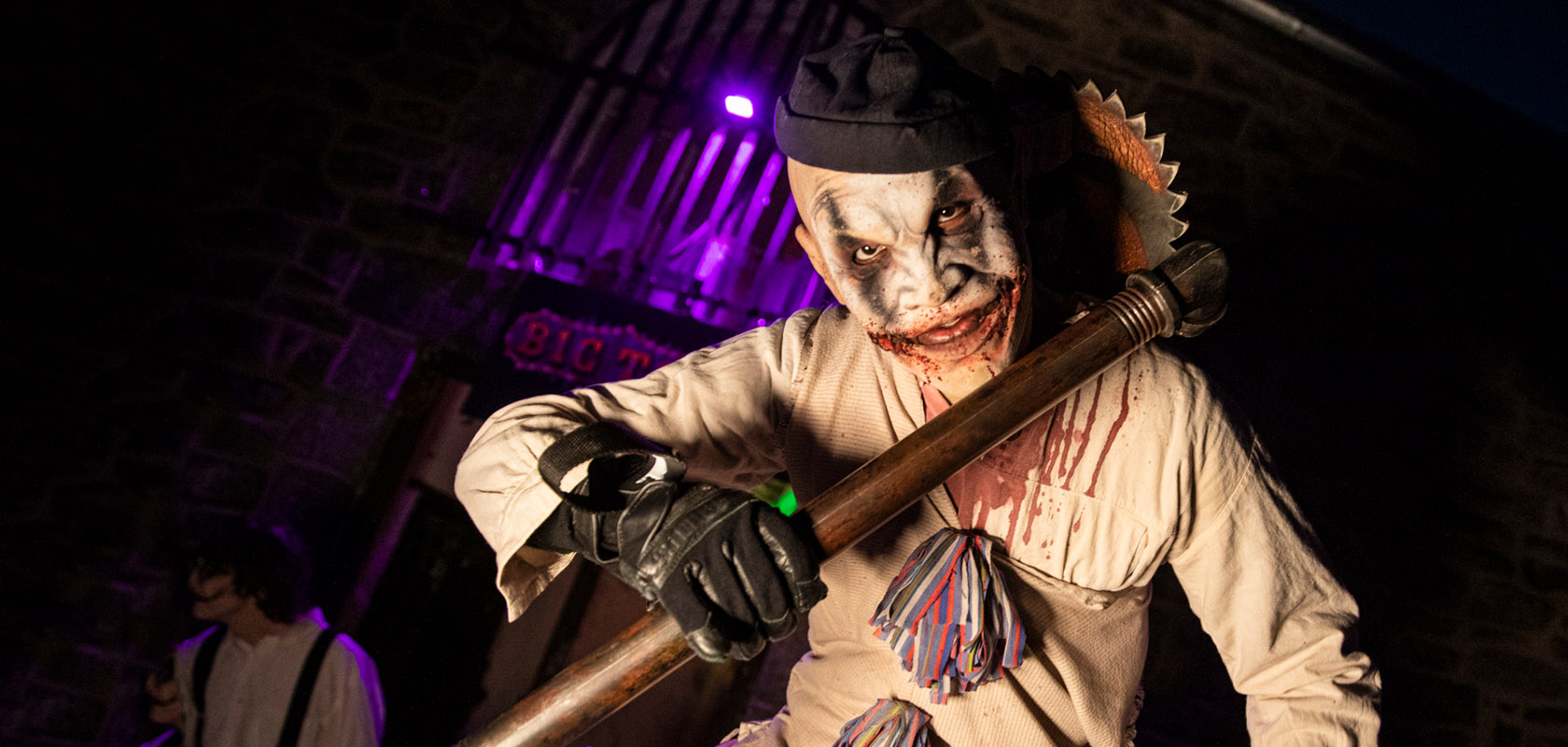The photograph shows two figures dressed in horror-themed or Halloween costumes amidst a dark and eerie setting. The main figure in the foreground is a terrifying character with a white face adorned with exaggerated makeup, featuring a wide, Joker-like mouth extending into his cheeks and black lines running from his eyebrows down to his mid-cheeks. He is dressed in a tan suit with large, ribbon-like buttons and is covered in bloodstains. He grips a long wooden pole, at the end of which is a menacing circular saw blade resting on his shoulder. He also wears black winter gloves.

In the left background, another male figure, less visible due to the darkness, wears a white shirt, black trousers, and suspenders, with a white, Joker-like face paint and long brown hair. A neon purple sign partially reading "BIG" is visible behind them, adding to the sinister ambiance. Both figures seem to evoke imagery from the movie "A Clockwork Orange" and project an unsettling, uncaring demeanor.